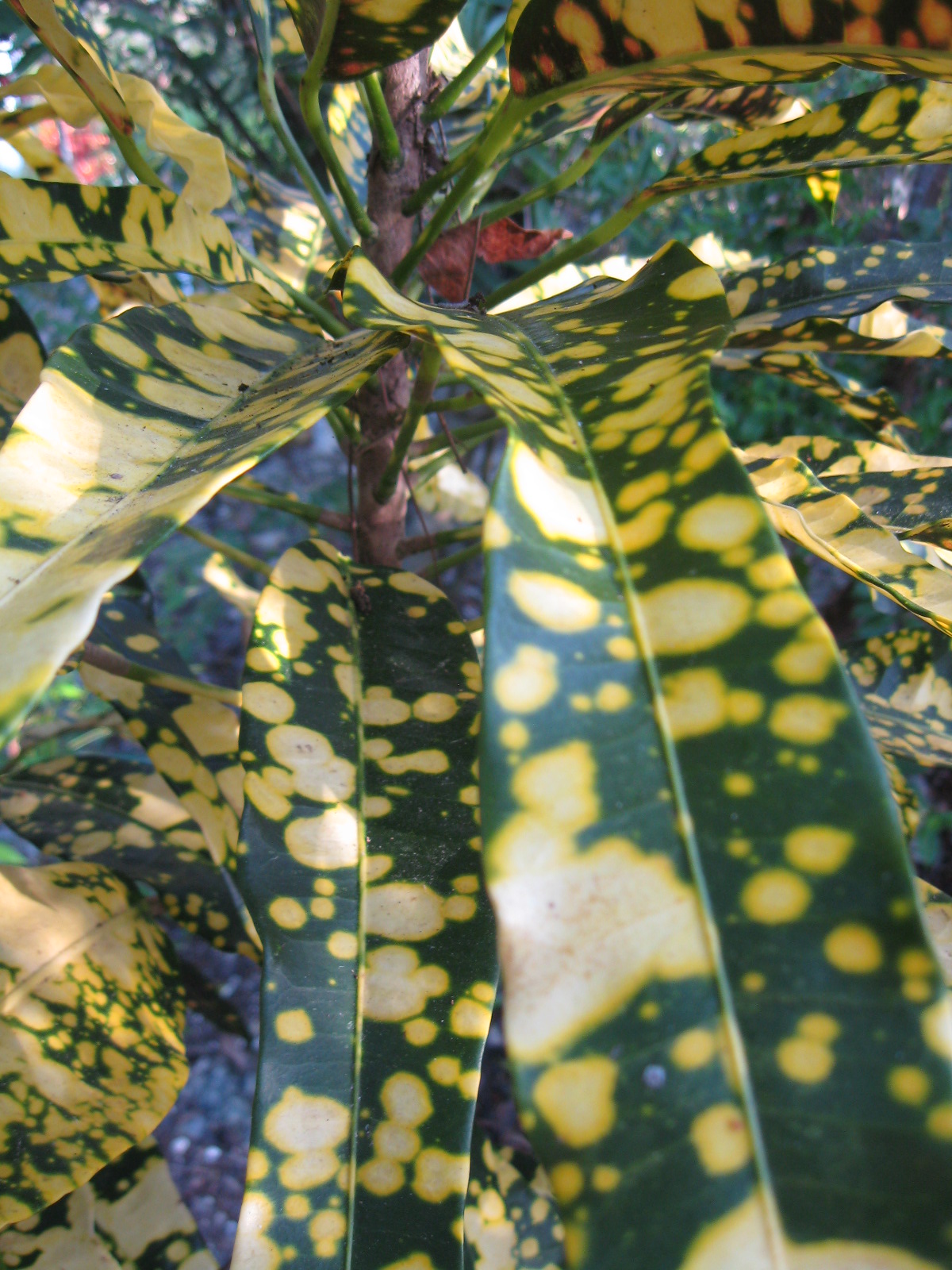This photograph captures a highly detailed, close-up view of a plant with long, dark green leaves prominently covered in yellow spots. Dominating the entire frame, the photo reveals a seemingly diseased or uniquely patterned plant with leaves extending outward from its center. On the right side, a single leaf nearly occupies the entire space, showcasing the intricate details of its unusual coloration. The background is slightly blurred, hinting at additional foliage and perhaps more trees. Some leaves even exhibit orange-red dots, adding to the surreal and almost computer-generated appearance of the plant. Overall, the image focuses intently on the striking, spotted foliage against the backdrop of a bright, sunny day.